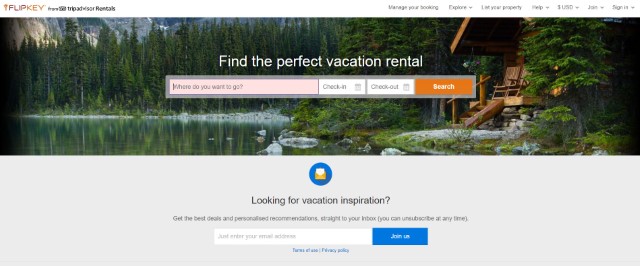Screenshot of the FlipKey rental website, displayed prominently at the top is a sleek white menu bar. On the left side, the bar features the FlipKey logo, a key icon, accompanied by the text "FlipKey" in elegant gold lettering, followed by the phrase “from TripAdvisor Rentals” in black. Beneath the menu bar is a scenic banner showcasing a picturesque lakeside setting, framed by a dense pine forest, and a charming wooden cabin nestled to the right.

Central to this tranquil outdoor image is a search bar inviting users with the prompt, "Where would you like to go?" Adjoined to the search bar are fields for check-in and check-out dates, followed by a search button. The header above the search bar reads, “Find the perfect vacation rental,” hinting at a world of possibilities. Below this inviting image, a gray section offers further engagement with the text, "Looking for vacation inspiration."